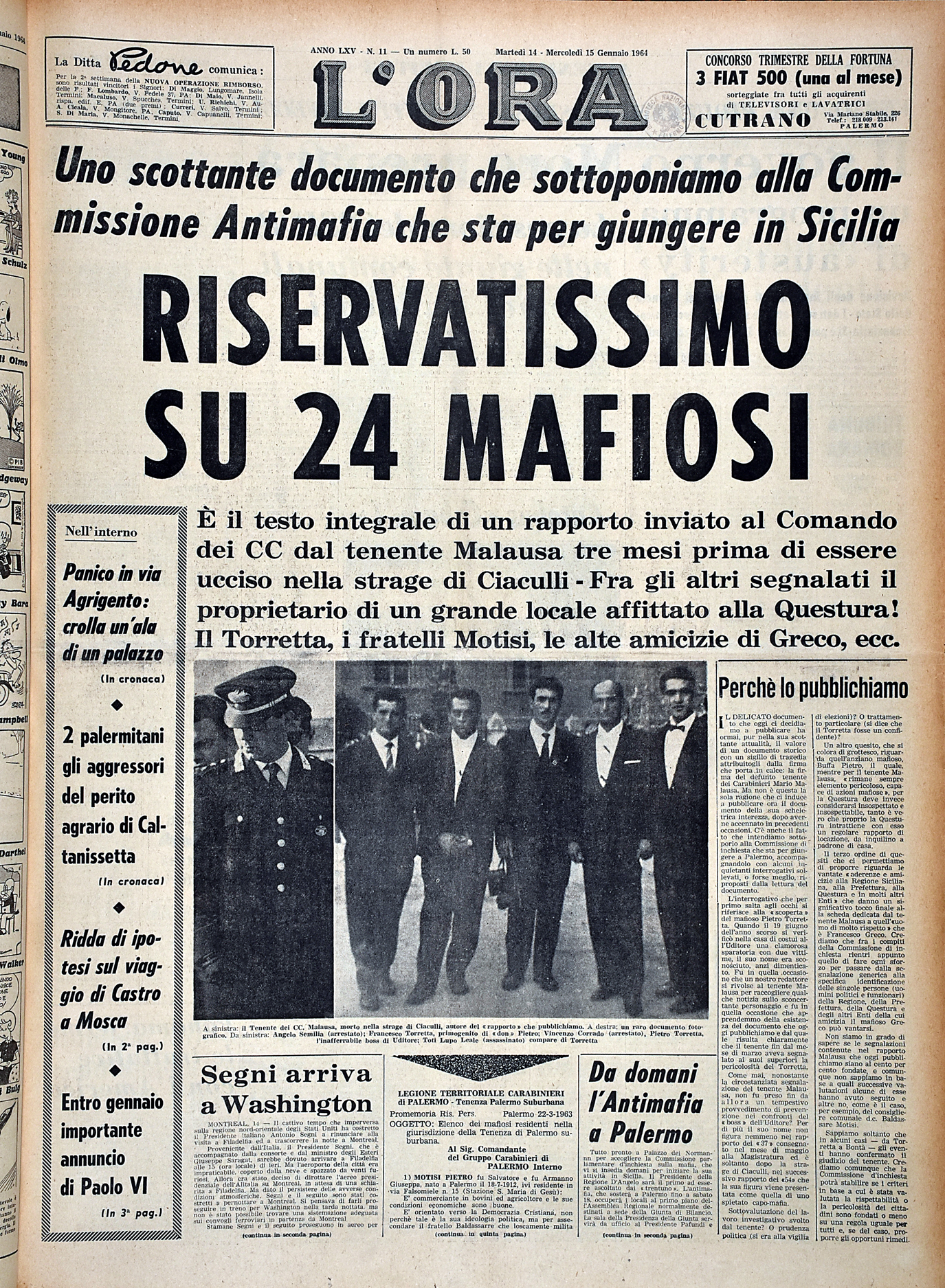This image is a clipping from a vintage Italian newspaper named L'Ora, dating back to 1964. The edges of the paper have yellowed with age, emphasizing its antiquity. Dominating the top third of the clipping, the headline "Riservatissimo su 24 mafiosi" suggests a confidential article focused on 24 members of the Italian Mafia. The text, written in Italian, includes phrases like "Uno scottante documento ci sottoponiamo alla commission antimafia che sta per girare in Sicilia," alluding to a sensitive document submitted to an Anti-Mafia Commission operating in Sicily. Central to the image are black-and-white photographs of five men in suits, alongside a police officer, likely relating to the mafia article. Additional side stories include references to Palermo and Washington, with a notable mention of Segni's arrival in Washington. The left-hand side features a block of text, possibly directing readers to other articles. An advertisement for Fiat adorns the top part of the clipping, adding to its historical context.